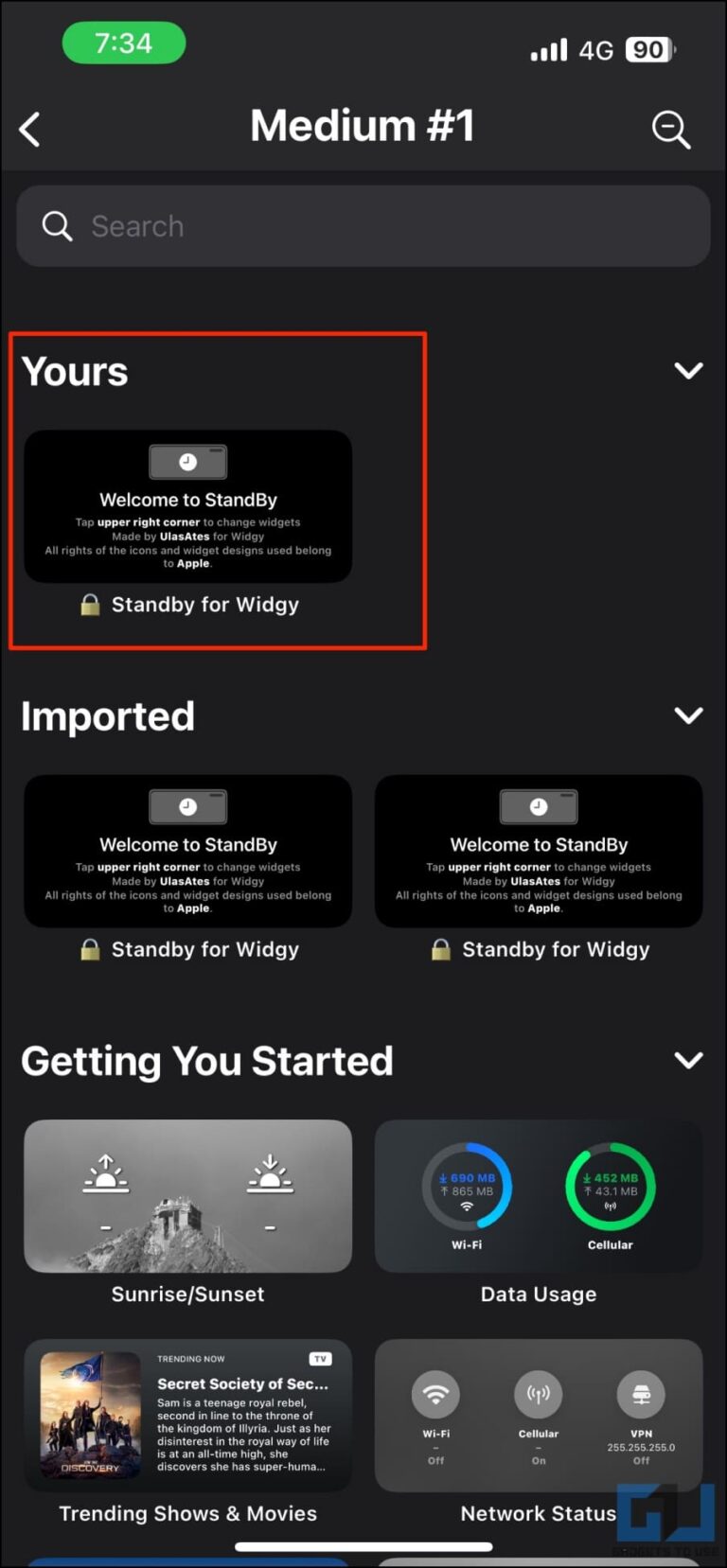A detailed caption for the provided image could be:

"The image depicts a screen from a mobile application interface showcasing multiple widgets and options. In the top left corner, a green battery icon indicates 90% battery life, accompanied by a 4G signal indicator with full bars. Centered at the top, the time is displayed as 7:34. The screen title, 'Medium 1,' is followed by sections titled 'Yours,' 'Imported,' and 'Getting You Started.' Within the 'Yours' section, a prominent red box highlights a widget labeled 'Welcome to Standby,' which includes instructions for changing widgets. The sections below display a variety of widget options, including sunrise and sunset times, trending shows and movies, data usage, and network status. The interface features a predominantly black background with white text, and the widgets are accented with various icons and graphics. In the bottom right corner, a watermark reading 'jjgj' is visible."